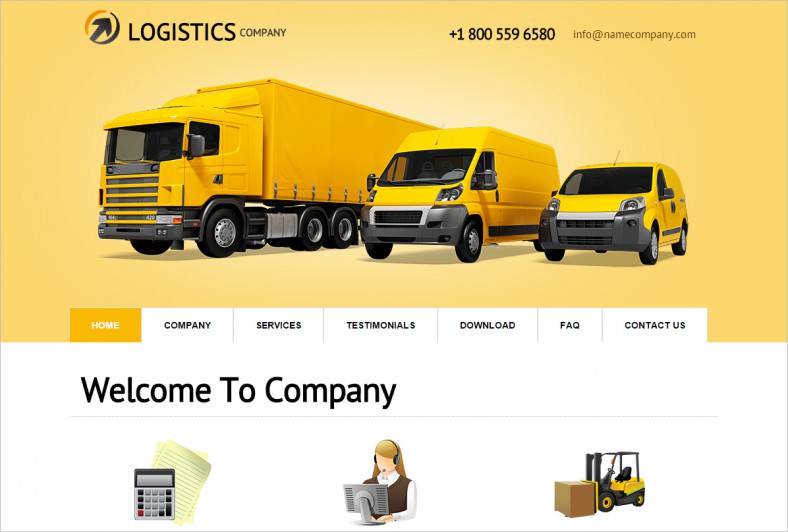This web page belongs to a logistics company and boasts a visually appealing design. At the very top, there's an image with a light yellow background featuring three bright yellow vehicles: a moving truck on the left, a moving van in the center, and an economy-sized van or SUV on the right. Just beneath this image, a menu bar with white tabs caters to easy navigation, offering options such as Home, Company, Services, Testimonials, Download, FAQ, and Contact Us. The selected tab is highlighted in yellow with white text for clear identification.

Below the menu bar, the header "Welcome to the Company" warmly introduces visitors to the site. Directly underneath this header are three informative icons: the center one displays a woman at a computer wearing headphones, representing customer support; the icon on the right depicts a forklift, symbolizing material handling; and the one on the left shows a stack of papers accompanied by a calculator, indicating administrative or financial services.